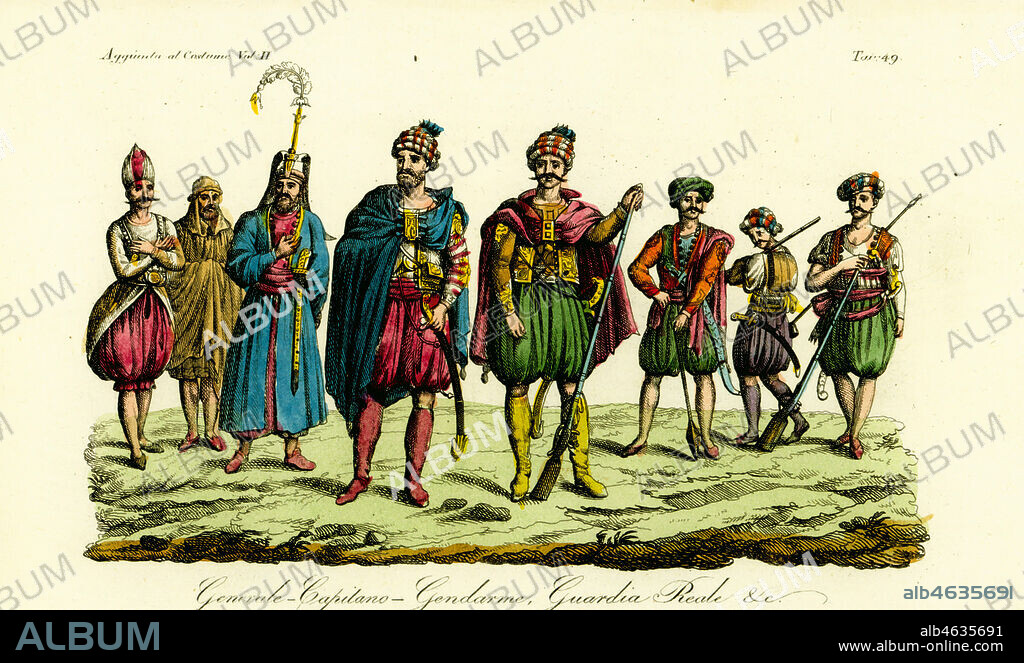The vintage illustration depicts eight men standing together in detailed and colorful Turkish costumes. The men are arranged with two in the foreground and three on each side, slightly in the background, all standing on a light green, grassy surface that resembles rock. Their attire is incredibly varied and vibrant, showcasing colors like green, yellow, red, orange, gold, brown, blue, cranberry, and dark purple. Some are wearing capes, tunics, robes, and possibly surcoats, accompanied by billowing breeches, knee socks, and shoes, while others appear to have bare legs. Each man dons unique headgear, such as woven turbans, and all have dark mustaches and dark hair tucked under their hats. Many of the men hold long rifles, giving a nod to medieval weaponry. The background of the illustration is a light parchment color, with the word "ALBUM" prominently printed diagonally across the image. In the lower left corner, it also reads "album," while the bottom right corner features the website www.albumonline.com along with a small number identifying the illustration. The artwork is rich with intricate details, including the folds and creases in the clothing and small cursive writing that is difficult to read.